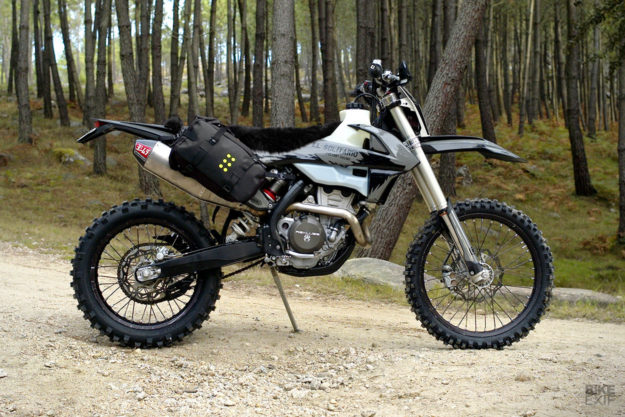In the image, a black and white dirt bike rests on its kickstand on a dirt path in a wooded area. The scene captures a serene outdoor setting, where evenly spaced, smooth tree trunks dominate the scenery, extending into the background without visible branches or leaves, giving an impression of stillness. Layers of brownish-green grass and weeds add a natural, somewhat wild feel to the ground beneath the trees. Scattered rocks, including a few large ones, dot the space behind the motorcycle, forming a rugged backdrop. The bike, which features thin black tires, a black seat that appears fuzzy, and a white body complemented by protective shields over the wheels, is photographed in profile, facing to the right. Attached to its side is a saddlebag adorned with golden buttons, adding a touch of practicality to its adventurous design. Through the myriad of tree trunks, a sliver of sky peeks through in the far background, suggesting a sunny day, while subtle greenery at the base of some trees hints at life amid the dormant woods.